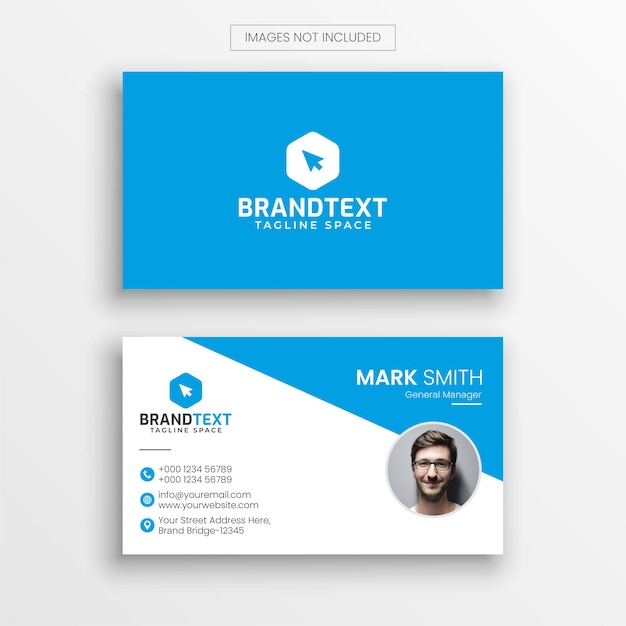The image features two sides of a business card template displayed against a white backdrop. At the top of the image, the text "images not included" is written. The top card showcases a bright blue background with a centered hexagon logo that reads "brand text tagline space" in white lettering. An arrow points up and to the left from the hexagon. The bottom card presents the completed front and back of the business card. The blue area on the right side displays the name "Mark Smith," his title "General Manager," and a circular photo of Mark—a young man with short hair, wearing glasses, and smiling at the camera. To the left, the business card includes the same "brand text tagline space" logo, along with icons for a phone, email, website, and address. The phone number is +000123456789, the email is info@youremail.com, the website is www.yourwebsite.com, and the address is listed as your street address here, brand bridge-12345. The overall layout serves as a customizable template for creating personalized business cards.